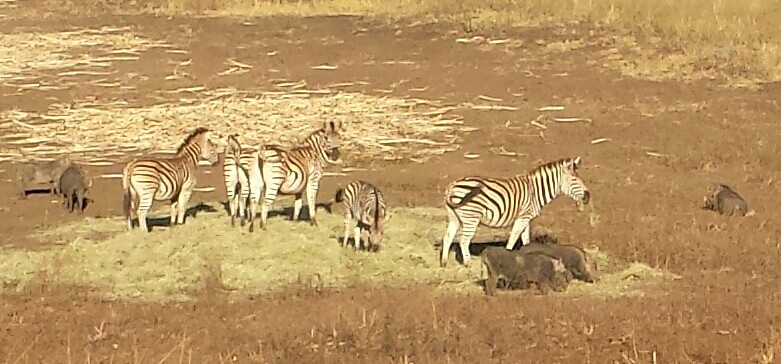The image depicts a group of five zebras and four wild boars, or warthogs, gathered on a patch of dry, yellowing grass that contrasts with the surrounding dirt terrain. The zebras, adorned in their characteristic black and white stripes, include an adult and its calf, the latter appearing to munch on the parched grass. Near the forefront of the image, two boars, brown in color, are also feeding on the grass, while a third boar stands on the dirt, its direction ambiguous. In the background, a thin line of browned grass stretches horizontally, with patches of hay interspersed throughout the scene. The zebras are arranged in various poses, some with their heads down, eating, while others have their hindquarters facing the camera. One zebra’s tail is noticeably raised and curving across its hindquarters. The boars, primarily gray and brown, are positioned among the zebras, with one boar lying down towards the right side of the image, making it difficult to discern its orientation.